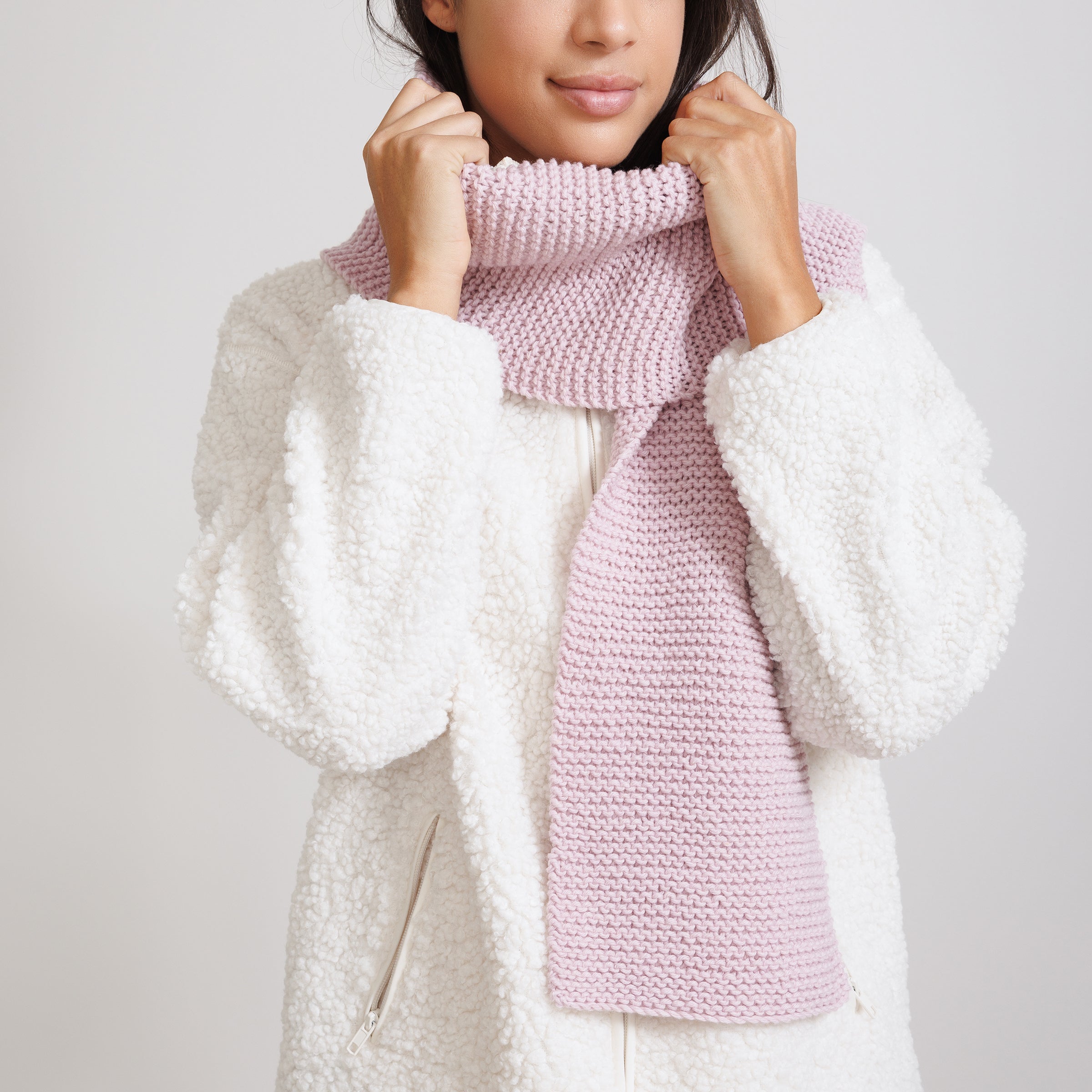This square color photograph features a model wearing winter attire, showcasing a mid-shot that frames her from the nose down, leaving out her eyes. She has dark brown hair and is wearing a wide, light pink knit scarf with a distinct, textured pattern wrapped snugly around her neck. Her full pink lips are accentuated by matching lipstick. She is dressed in a soft, white, fleecy sweatshirt that has a zipper down the front and two zippered pockets on each side. Both of her hands are positioned just under her chin, holding her scarf. The background is a uniform light gray, enhancing the focus on the model and her winter clothing. There is no text present in the image.